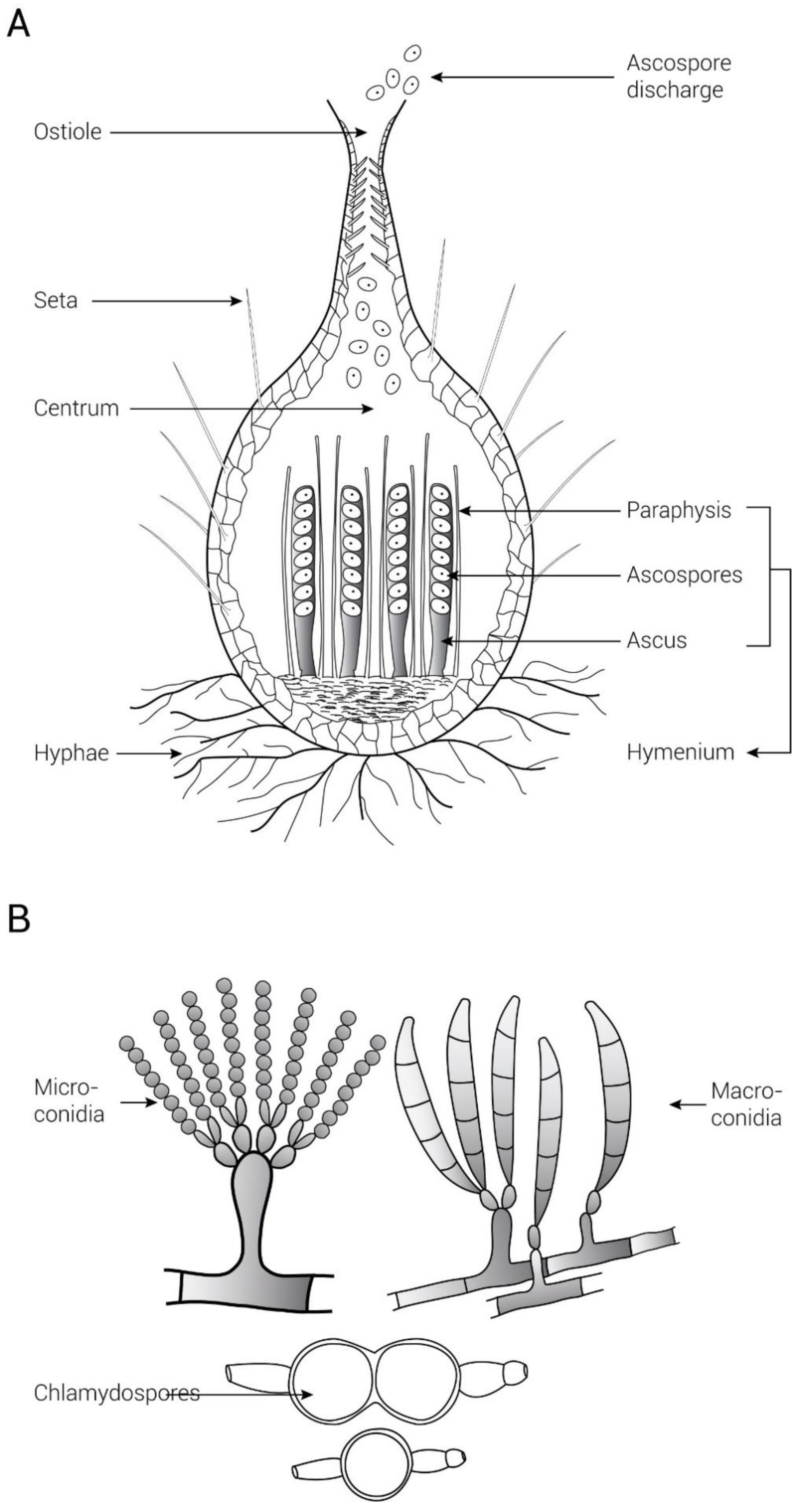This image is a black-and-white scientific drawing, likely from a scientific or plant biology book, displaying detailed diagrams labeled as 'Part A' and 'Part B'.

In Part A, the drawing depicts an oval-shaped structure resembling a plant root system. At the top, an opening labeled "Ascospore Discharge" shows spores being released. Surrounding this are various labels pointing to specific parts: "Ostiole" at the opening, "Centrum" in the middle section, and "Hyphae" at the base, where root-like structures appear. Additional labels include "Paraphysis," "Ascospores," "Ascus," and "Hymenium," all key components of the structure.

Part B features two separate illustrations of spore formations. On the left, labeled "Microconidia," is a detailed depiction of smaller spores. On the right, labeled "Macroconidia," shows larger spores. At the bottom, another label identifies "Chlamydospores," suggesting these are stages or types of spore development. This chart collectively outlines various structural and developmental aspects of plant or fungal biology.